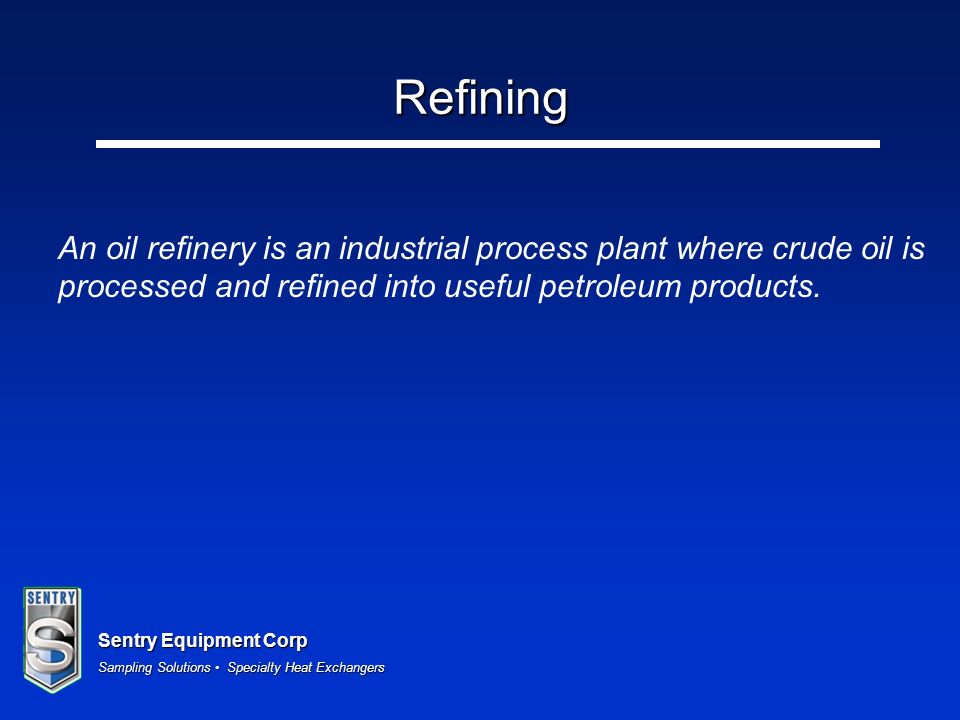The image depicts a blue PowerPoint slide with a graduated color scheme, transitioning from a dark navy blue at the top to a bright royal blue at the bottom. At the top center, in white block letters, the word "Refining" is prominently displayed, underlined with a thick horizontal white line. Below the underline, in white italics, the text reads, “An oil refinery is an industrial process plant where crude oil is processed and refined into useful petroleum products.” Positioned in the bottom left corner is a logo with quadrants of blue and grey, featuring a large grey letter 'S' and the word "Sentry" in blue letters. To the right of the logo, in blue block letters, it states "Sentry Equipment Corp," followed by smaller white text that reads, “Sampling Solutions. Specialty Heat Exchangers.”